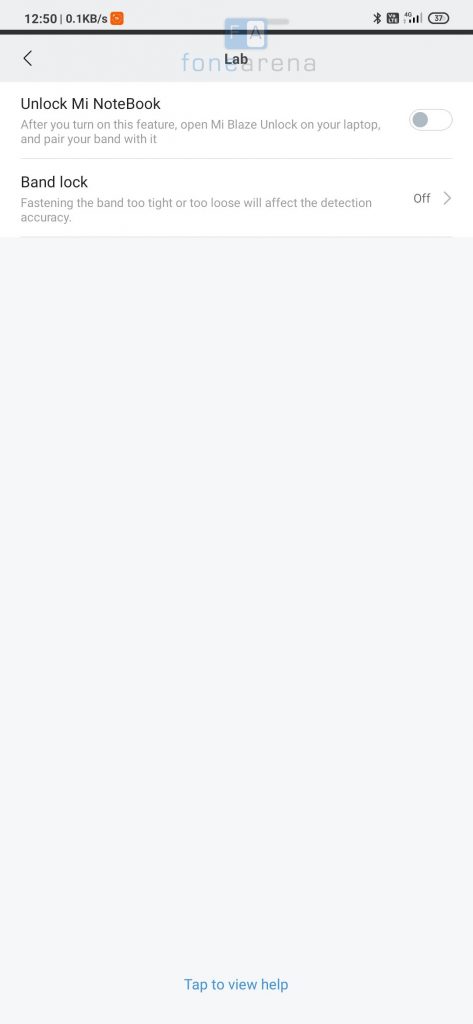Here is a cleaned-up and detailed caption for the described image:

---

The screen capture of a mobile device displays a page from an app called “FoneArena.” At the top center of the screen, there is a watermark featuring a blue rectangle with a stylized "S" on the left and an "A" on the right. The "A" is blue with a white background, while the "R" next to it is white with a blue background. Just below the watermark, the text appears to read "FoneArena" or potentially "FoneC," though the last letter is unclear.

Below the watermark, the page is labeled "Lab." On the top left corner is a back button, represented by a caret symbol (less than sign "<"). The main section of the page starts with a heading that reads, “Unlock Mi Notebook,” which seems to be a feature instruction. The text below it states, "After you turn on this feature, open Mi Blaze Unlock on your laptop and pair your band with it." To the right of this instruction is a toggle switch that is currently set to off.

Further down, another setting is labeled "Band Lock," with a description reading, “Fastening the band too tight or too loose will affect the detection accuracy.” This setting's toggle switch is also turned off. At the very bottom of the page, there is a button labeled "Tap to view help."